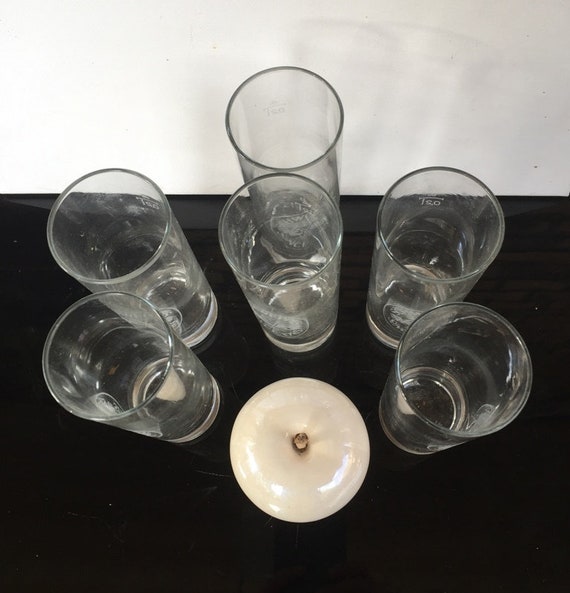The photograph captures a bird's eye view of a black matte table set against a plain white background, possibly suggesting an indoor setting given the faint shadows cast by the objects. Six tall, straight drinking glasses, each containing a few centimeters of water, are arranged symmetrically on the table. Two are positioned in the top left corner, two in the top right corner, and two more vertically aligned above a central object. While some glasses display smudges and fingerprints, adding a sense of use, a single glass teeters precariously at the edge of the table. In the middle of the composition lies a white object, resembling an apple, further alluding to the possibility of the photograph being black and white despite initial perceptions of color. The overall composition, with its crisp details and careful arrangement, creates a striking visual that emphasizes the simplicity and subtle imperfections of everyday objects.